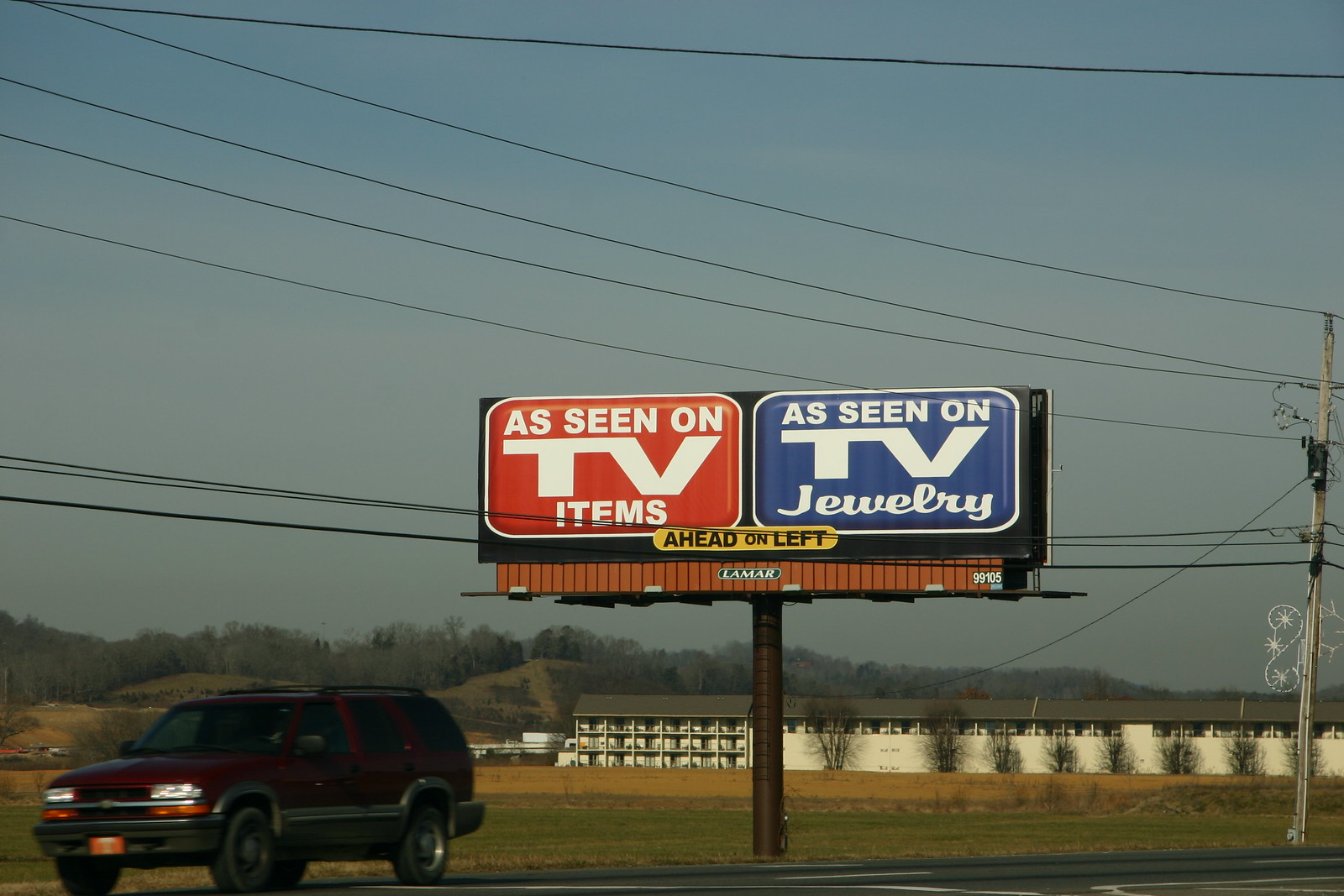The image features two enormous billboards prominently positioned in a vast, open field adjacent to a roadway. The billboards stand side by side, each affixed atop a massive, rectangular-shaped brown pole deeply embedded into the grassy area. The first billboard, striking in red with bold white lettering, advertises "As Seen on TV Items." In contrast, the second billboard, entirely blue, promotes "As Seen on TV Jewelry" and features a smaller sign underneath that reads "Ahead on Left." The extensive and detailed visual presentation highlights the commanding presence of the billboards against the expansive, natural backdrop, drawing the viewer's attention to their messages and directions.